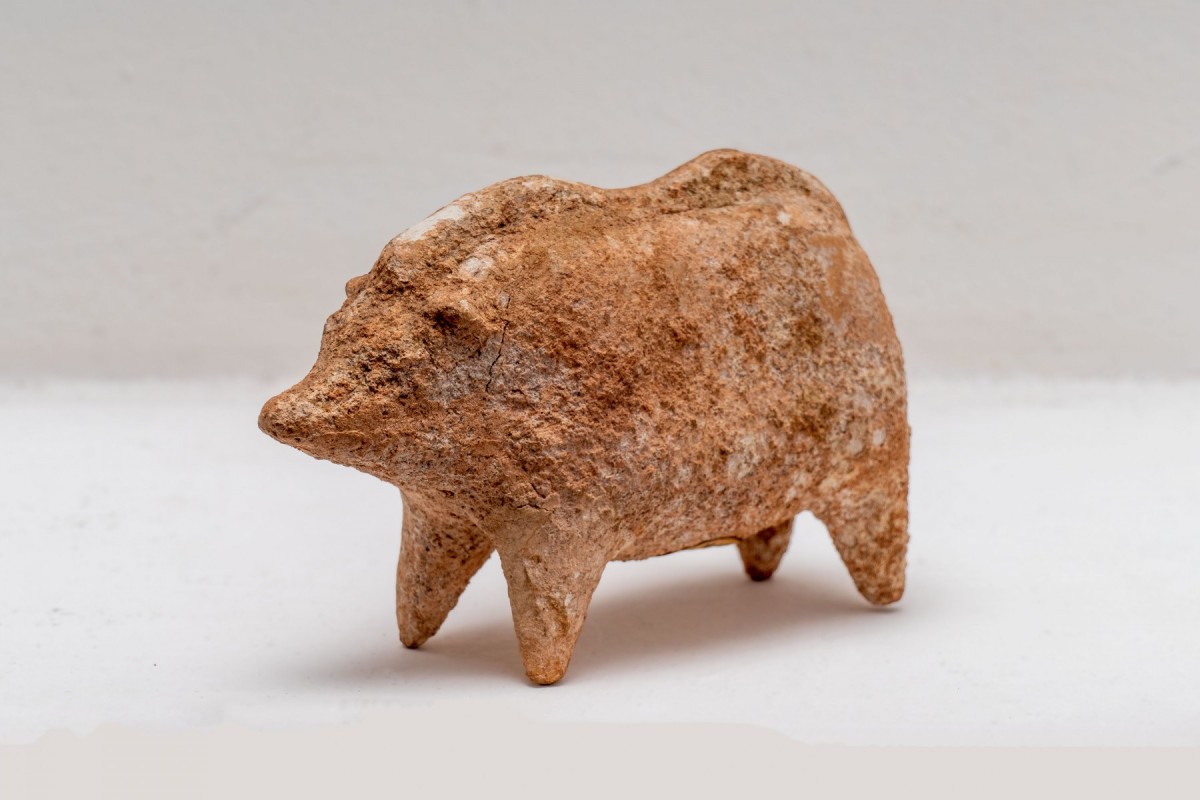The image showcases a close-up photograph of an ancient terracotta-colored ceramic sculpture, likely from a museum collection, set against a white background. The surface is brightly illuminated, with shadow making the white background appear slightly darker. The piece is a simplistic yet robust depiction of an animal, possibly a pig, wild boar, or peccary. The sculpture features a large, rounded body supported by short, inverted cone-shaped legs, reminiscent of ancient Mexican art. The animal faces left, with noticeable short, pointy ears and a prominent snout. A defining ridge runs from the top of its head to its back. Despite its minimalistic design, you can make out the eye on the side facing the camera, along with a small crack just behind the ear.